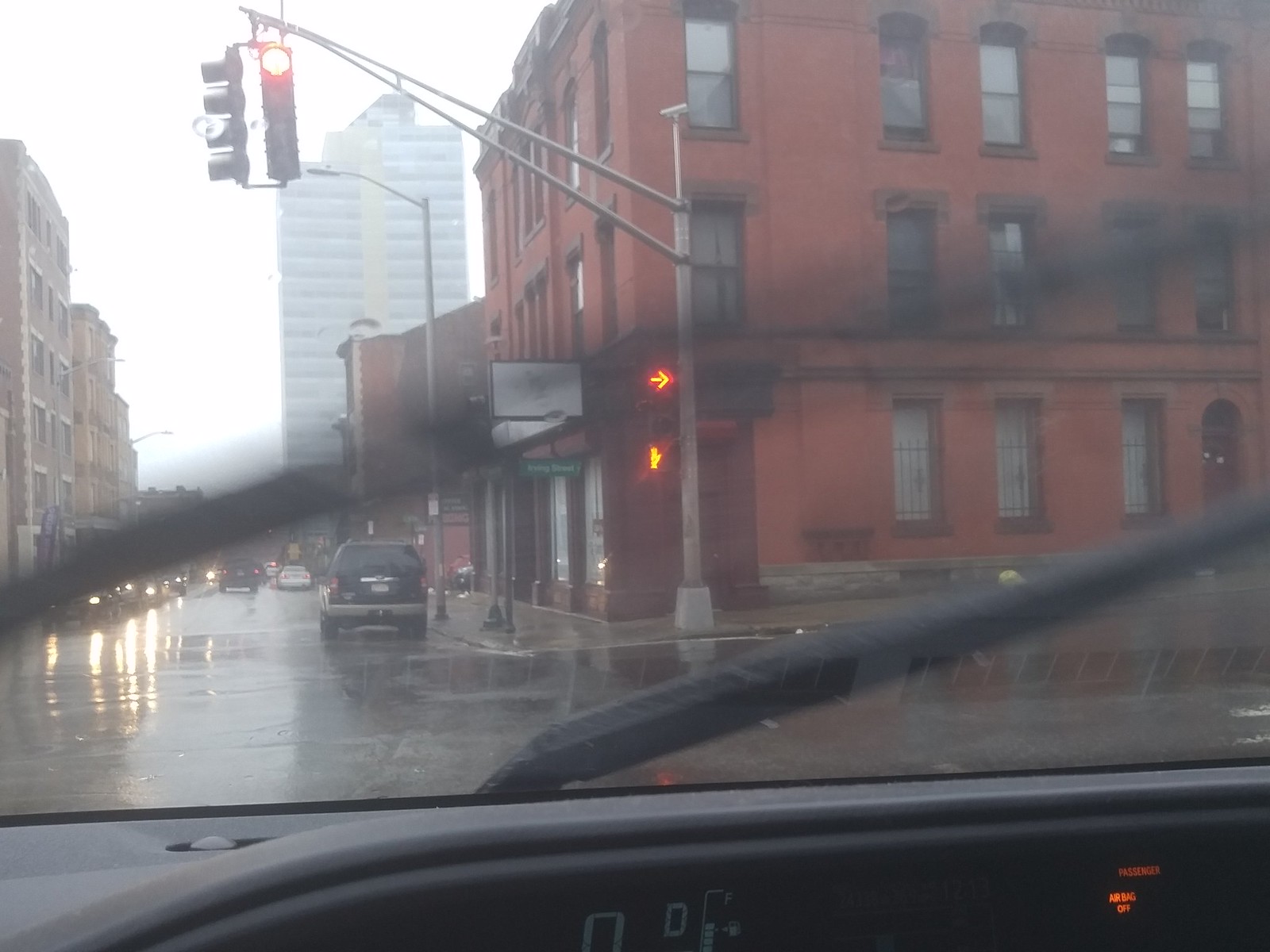In this color photograph taken from the driver's seat of a car, the view extends through a rain-speckled windshield, catching the mid-sweep of the windshield wipers. The scene captures a rainy city intersection as the car waits at a red light. Directly across the street, a large, imposing brownstone building stands at a corner, marked by a sign with an arrow pointing to the right and another sign below it emitting a bright orange light. In the background, a towering skyscraper looms, its height accentuated against the overcast sky. To the left side of the image, various smaller buildings line the street, accompanied by several parked cars and others waiting with their headlights on. Street signs punctuate the scene, contributing to the urban landscape. The rain-soaked pavement enhances the melancholic, muted colors of the surroundings, with puddles reflecting the city's lights and structures.